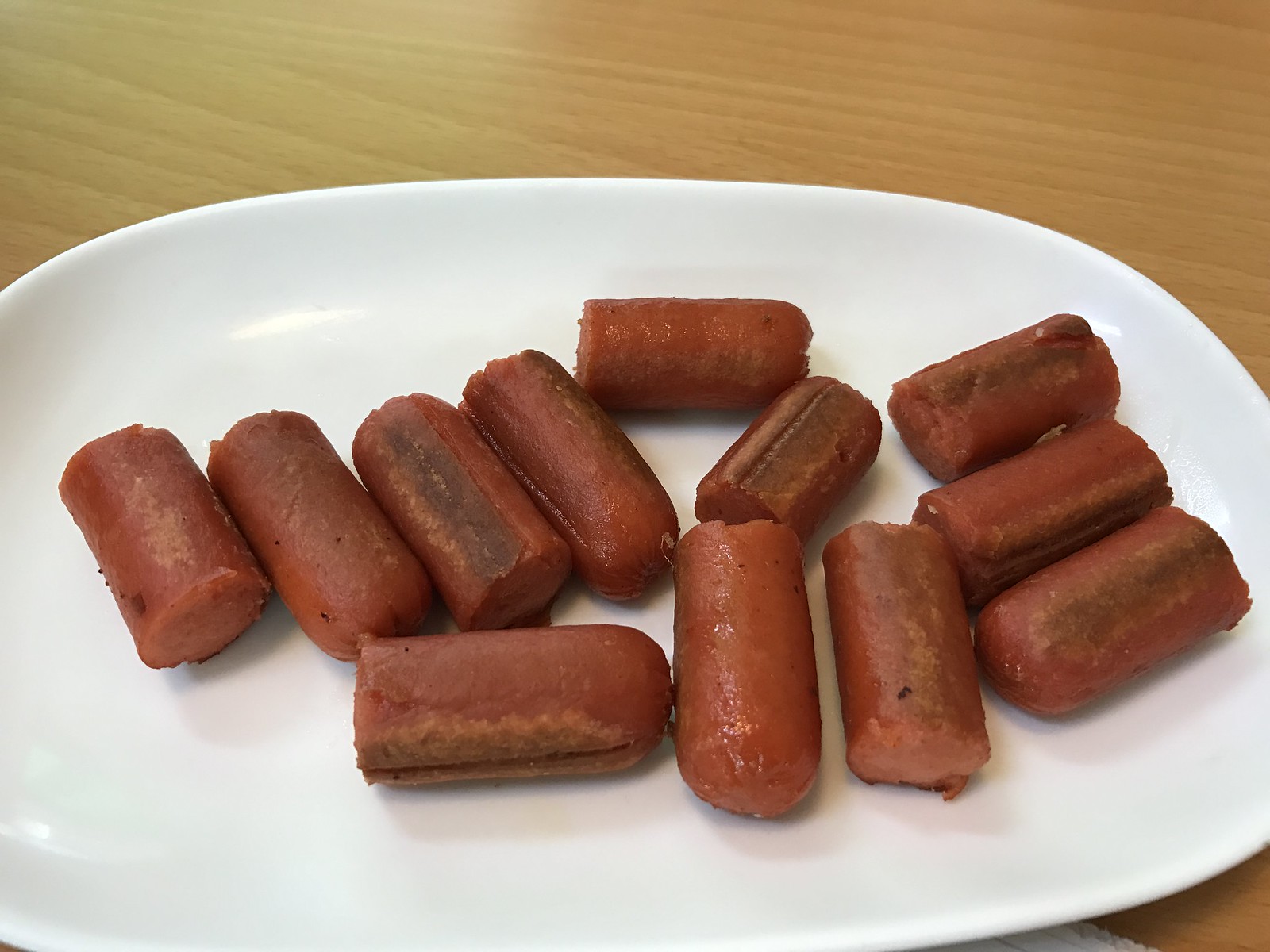In this close-up image, a white, elongated oval ceramic plate is set against a blonde-colored wooden surface, likely a veneer-style top with visible grain patterns. The plate contains 12 neatly sliced pieces of hot dogs, each browned and crisp on the exterior, suggesting they were either fried in a pan or grilled. The hot dog slices vary slightly in size and shape but are consistently similar overall, resembling the size of baby carrots. The surface they rest upon has an understated, casual charm that complements the rustic presentation of the well-cooked, char-marked hot dogs.